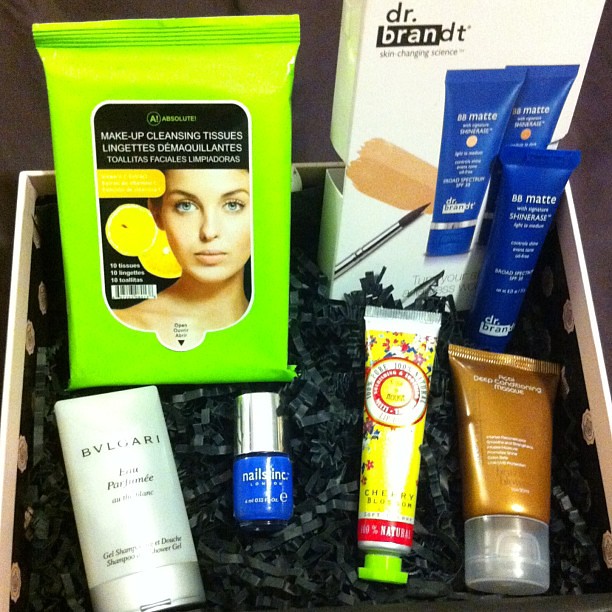This detailed photograph showcases an open gift box filled with various personal care and cosmetic items, set against a dark background. The brown box, adorned with small polka dots, is lined with crinkled black paper fillers. Prominently among the contents is a bright green package of Makeup Cleansing Tissues featuring a woman's face and lemon slices, located at the top left. To the top right of the box is a white square container labeled "Dr. Brandt," containing blue tubes of skincare products. Below this, a wide bronze-brown shimmery tube with a clear cap sits next to a bright yellow skinny tube, identified as a conditioner. 

At the bottom left, there is an elegant white oblong tube by Bulgari, capped with silver. Adjacent to it is a small blue glass bottle of nail polish with a silver lid. Additional items include a tube of makeup with a red and yellow design indicating "cherry blossom" and another slim blue tube situated just above the "Dr. Brandt" label. The collection of products presented in this neatly arranged gift box emphasizes an array of skincare and cosmetic essentials, all meticulously photographed to highlight their vibrant colors and detailed packaging.